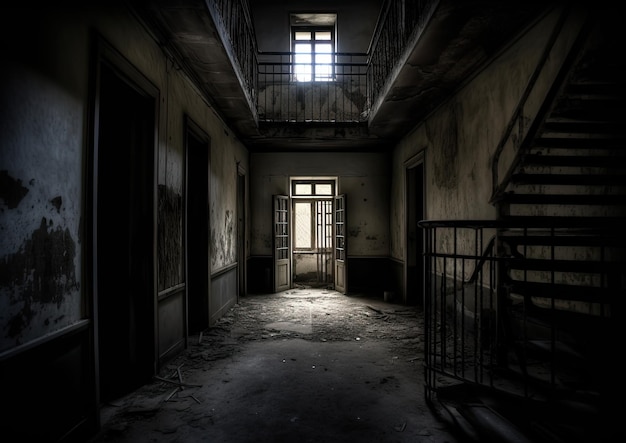The image depicts an interior shot of an abandoned, dilapidated two-story building. The scene is centered on a dark gray concrete hallway littered with broken wood, dust, and dirt. The hallway's walls are adorned with light-colored wallpaper marred by numerous brown stains and torn patches. On the left side of the hallway, there are three doorways, with the third located at the very end. At the end of the hall, French doors open into a back room illuminated by a window, the sole light source. The right side of the hallway features a single doorway located further down the hall. In the foreground's bottom right corner, a black staircase with visible railing ascends to the right and out of the image. The second story is visible and features a railing around an open central area, forming a walkway along the upper walls. The upper floor has a white wall and another window emitting bright white light, contributing to the overall worn and neglected aesthetic of the building.